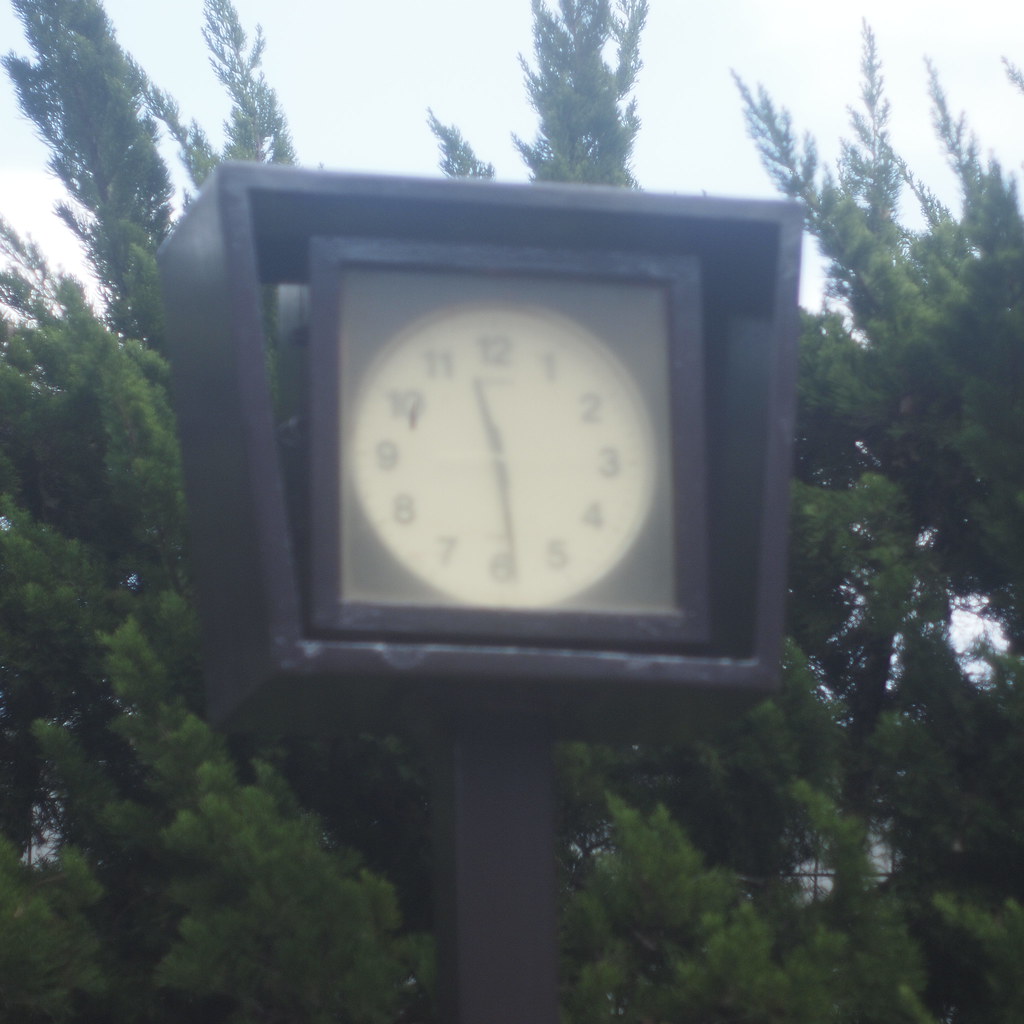This photograph depicts a street clock mounted on a signpost. The signpost appears to be black, possibly made of cast iron, and is topped with a square frame that encloses the clock. The frame itself is black and contains another smaller black metal box. Within this box is the clock face, which is round and white with bold, black numbers ranging from 1 to 12. The clock hands—black minute and hour hands—point to approximately 11:29. The glass covering the clock face appears foggy, slightly obscuring the view. In the background, there is an overcast gray sky and several evergreen trees, their needle-like leaves creating a dense backdrop behind the clock. The image appears to be slightly blurry, adding to the overall muted ambiance of the setting.